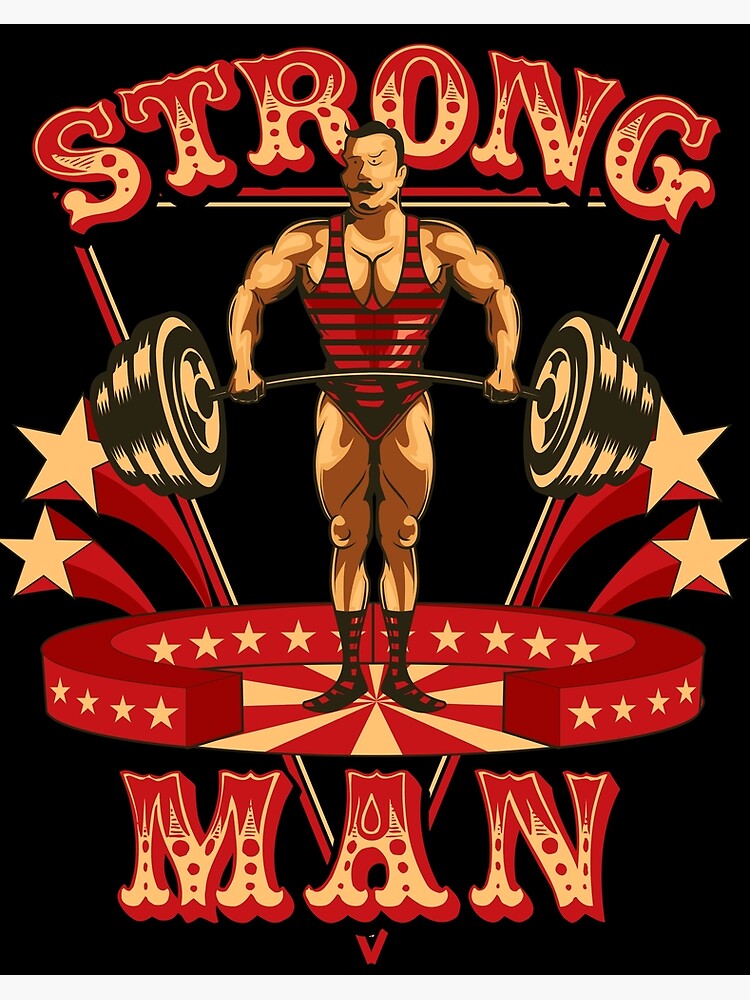This painting features a man standing at the center against a stark black background, exuding an aura of strength and determination. He stands atop a multicolored platform that combines red and beige elements, bordered by a small wall decorated with red and beige-colored stars. The man is clad in a striking one-piece outfit, reminiscent of vintage swimsuits, with a vibrant red base and bold black horizontal stripes accentuating his physique. His appearance is characterized by short black hair, a distinctive black mustache, and a small patch of black hair on his chin, adding to his robust demeanor. He confidently holds a barbell with sizable weights on each end, showcasing his musculature and power. The painting is framed by the words "STRONG" at the top and "MAN" at the bottom, both rendered in red letters with a subtle cream gradient at the lower portion, emphasizing the theme of strength and fortitude.